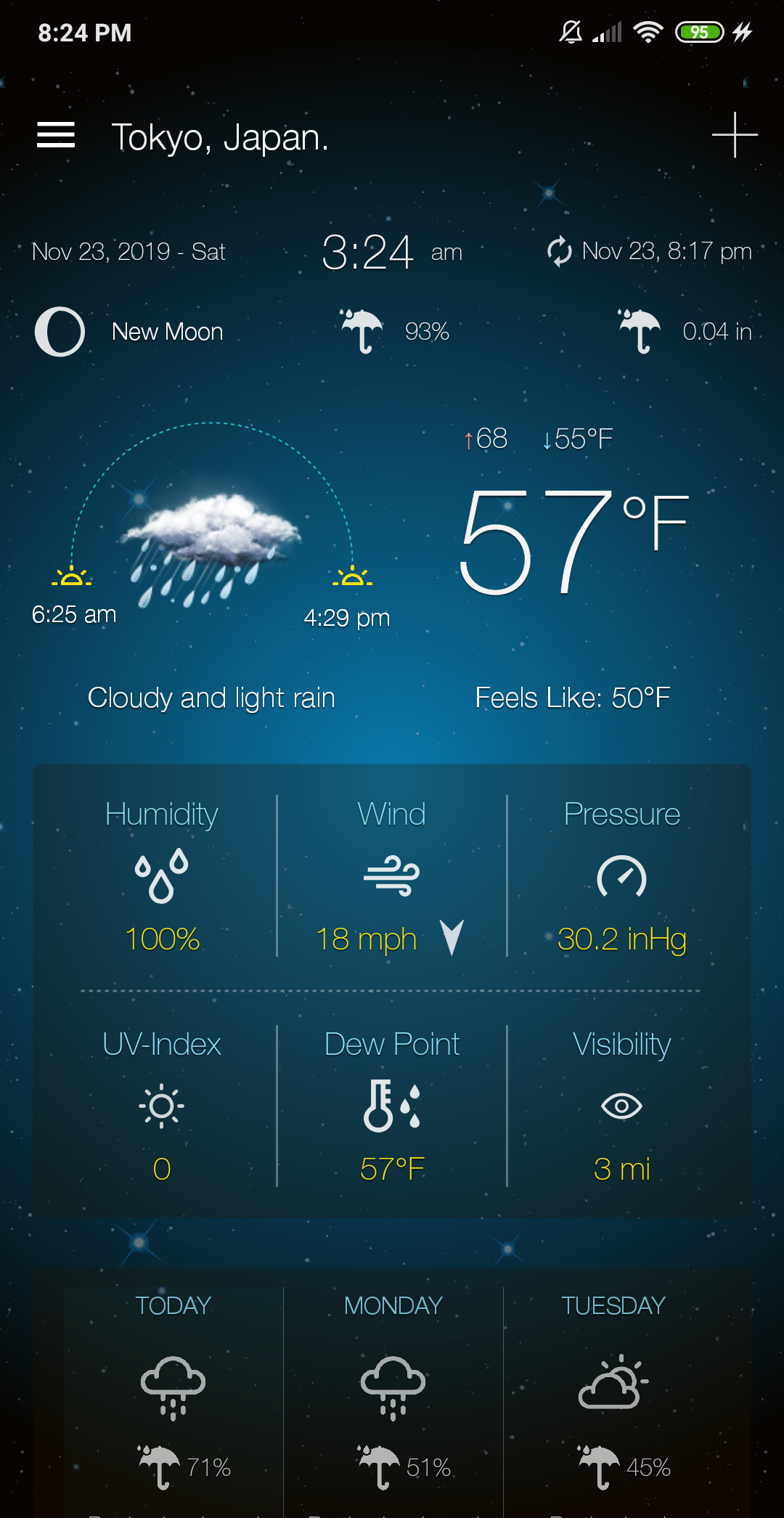The image features a detailed display of a weather application with a night sky background that fades from darker at the top to lighter towards the bottom. 

**Top Section:**
- **Top left:** 8:24 PM
- **Top right:** A bell icon with a line through it, followed by Wi-Fi signal bars, two of which are white and three are grey.
- A green rectangle containing "95" and two lightning bolt icons, encased in a white-outlined, bulging rectangle.
- Below this, a section displaying:
  - **Left:** Three horizontal lines with "Tokyo, Japan" written to the right.
  - **Right:** A plus sign, a date, and the time 3:24 AM.
  - A partial circle made of two arrows, another date, and a bow-like icon thicker on the left side, indicating "new moon."

**Middle Section:**
- An umbrella icon with raindrops, labeled "93%," followed by another umbrella icon labeled "0.04 IN."
- A cloud with raindrops, flanked by suns on either side, with a curved dotted line between the suns:
  - Below the first sun: 6:25 AM
  - Below the second sun: 4:29 PM
  - Below the cloud and sun icon: "Cloudy and light rain."
  - **Red dot:** 68°F
  - **Blue dot:** 55°F
  - Below the red and blue dots: 57°F, "Feels like 50°F."

**Measurement Section:**
- A blue rectangle labeled "Humidity" with raindrops icon: 100%
- A line separating sections, followed by "Wind" with a wind symbol: 18 MPH (arrow pointing down).
- Another line, then "Pressure" with a gauge icon: 30.2 INHG.
- A dashed line, then "UV Index" with a sun icon: 0.
- Another line, then "Dew Point" with a thermometer and drops icon: 57°F.
- Last line, "Visibility" with an eye icon: 3 MI.

**Bottom Section:**
- A darker blue rectangle labeled "Today" showing a cloud with raindrops and an umbrella: 71%.
- A line, followed by "Monday" with the same icons: 51%.
- Another line, followed by "Tuesday" showing a cloud with the sun and an umbrella: 45%.

Overall, the image is a comprehensive weather forecast for Tokyo, Japan, featuring current weather conditions, temperature, humidity, wind speed, pressure, UV index, and visibility. There are also short-term forecasts for the upcoming days.